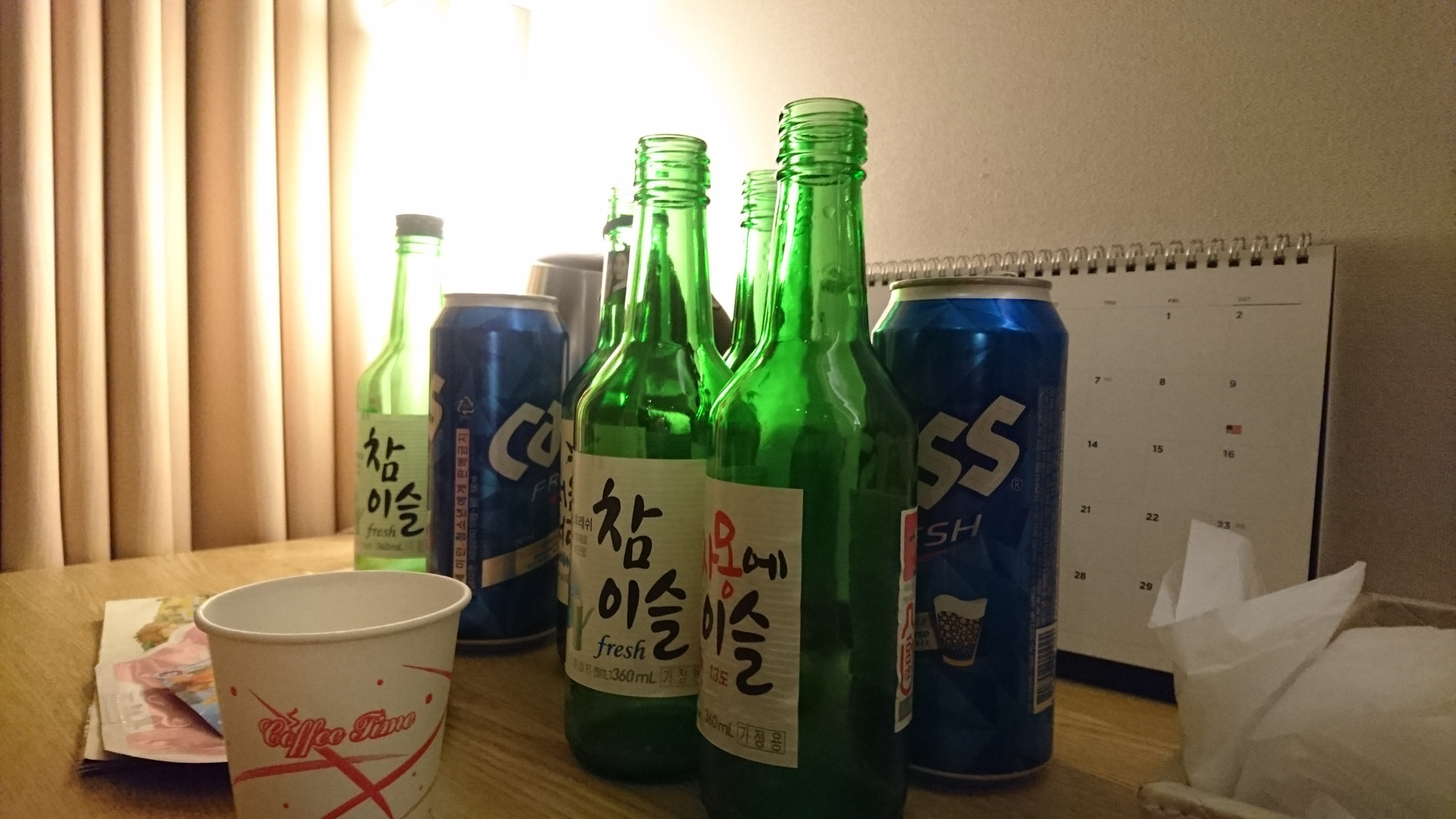The photo captures a lively, somewhat messy scene of someone's Friday night in a hotel room. Centered on a wooden table top, the main attraction is five empty green bottles of soju, their white labels adorned with Asian characters. Accompanying the soju bottles are two tall, blue cans of Cass beer, a popular South Korean brand. Positioned to the left of the bottles is a white coffee cup with the words "Coffee Time" in red, likely repurposed as a mixer for creating the beer-soju cocktail known as "so-mak." To the right, a small stack of tissues adds to the casual, lived-in feel of the setting. The backdrop features a closed tannish-salmon curtain illuminated by a nearby white light, adjacent to a plain tan wall. Leaning against this wall is a white calendar with black text, adding to the personal, intimate atmosphere of the room.